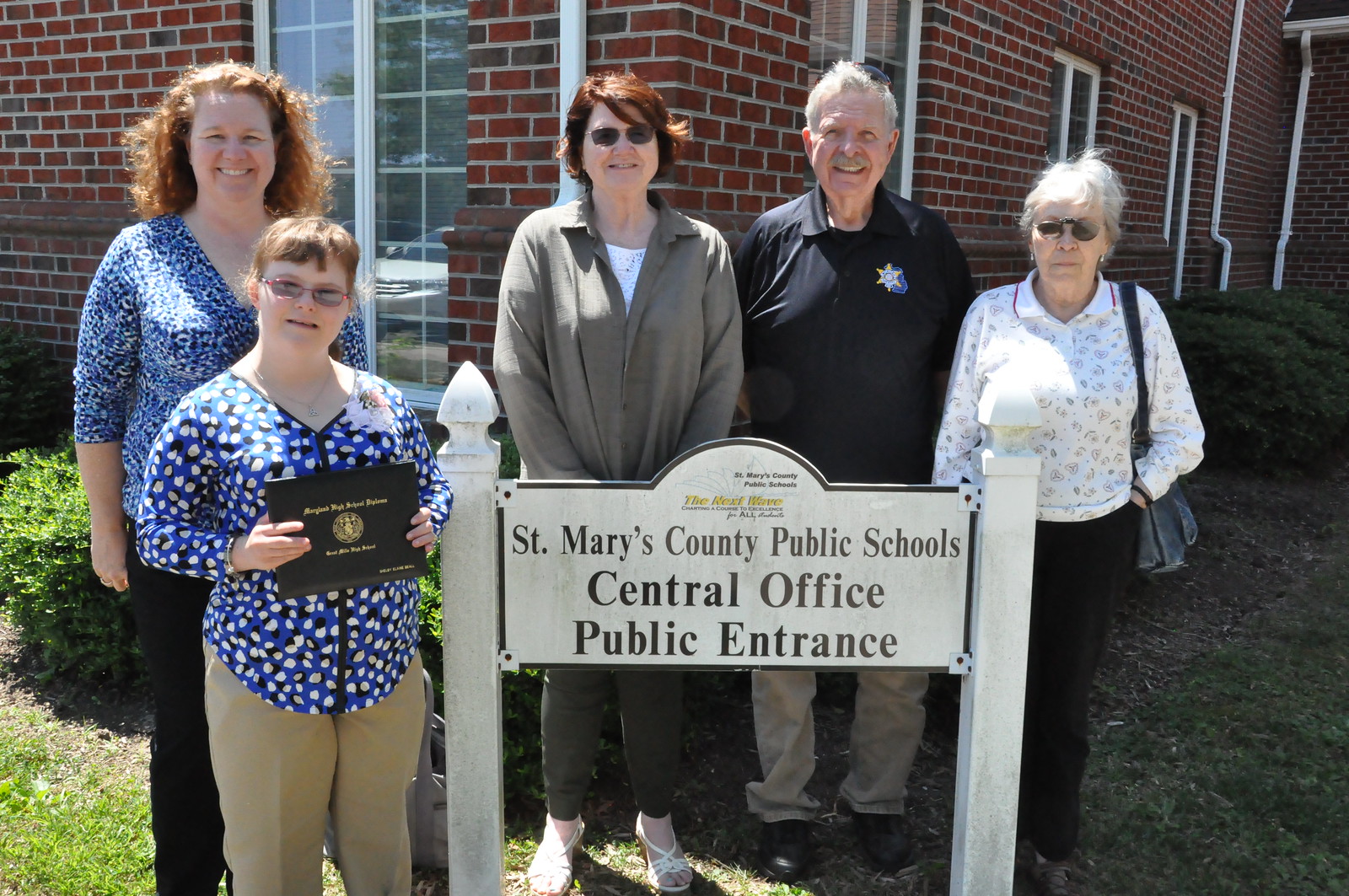In front of a red brick school building with tall segmented windows, a group of five people stands on a grassy area with green shrubbery behind them. Central to the scene is a white sign mounted on two white posts, though aged and in need of repair. The sign reads "St. Mary's County Public Schools, Central Office, Public Entrance," with "St. Mary's County Public Schools, the next wave" in yellow at the top.

On the far left are two individuals wearing blue blouses; the shorter one in front has glasses and beige pants. Centered behind the sign, a woman with red hair, glasses, and a gray jacket stands beside a man dressed in a black shirt and beige khakis. To their right, a much older woman, distinguishable by her white shirt, sunglasses, and a purse on her left arm, completes the group.

Prominently featured is a young girl in the front, proudly holding a black award or diploma case with gold lettering, hinting at a celebratory occasion, possibly a graduation. All five individuals are smiling, capturing a moment of shared joy and achievement.